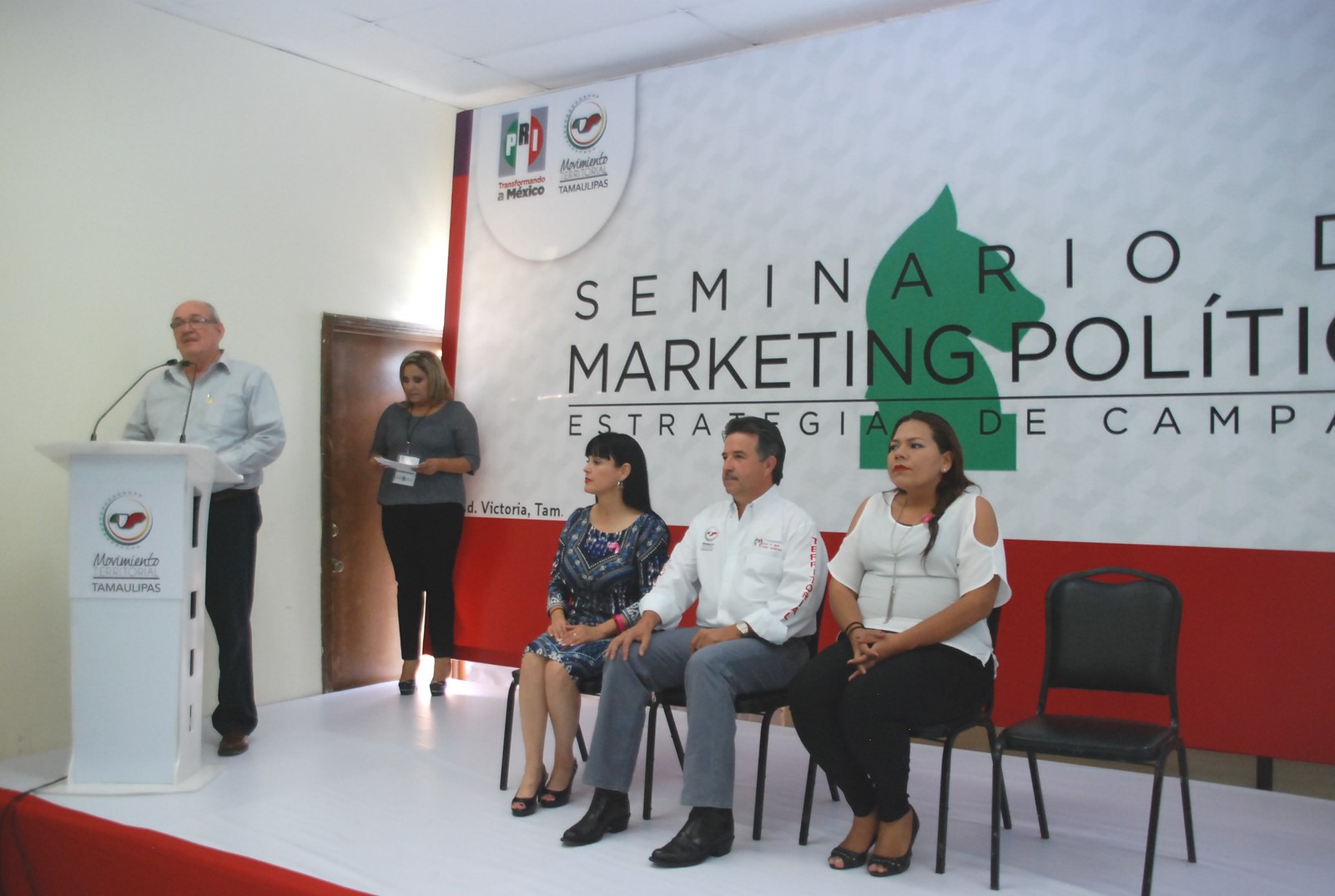The image depicts a stage setup for what appears to be a seminar, press conference, or university lecture. The stage floor is white, bordered by red front and back walls. A large white banner hangs on the red back wall, prominently displaying partially visible text in Italian, including the words "Seminario," "Marketing," "Politi...," and "Estrategia de Camp." Centered on the banner is an image of a gray horse.

On the left side of the stage stands a man dressed in a white button-down shirt and black pants. He is speaking into a thin microphone, hands positioned on a white podium, which bears the sign "Movimiento Tamaulipas." Behind him stands a woman in black pants and a gray sweater. She has blonde hair, is wearing high heels, and is holding a piece of paper, appearing to review its contents.

To their right are four chairs, three of which are occupied. The individuals seated seem somewhat apprehensive, their focus likely directed toward the unseen audience. This well-organized setting clearly indicates a formal event, with careful attention to visual details and professional attire.